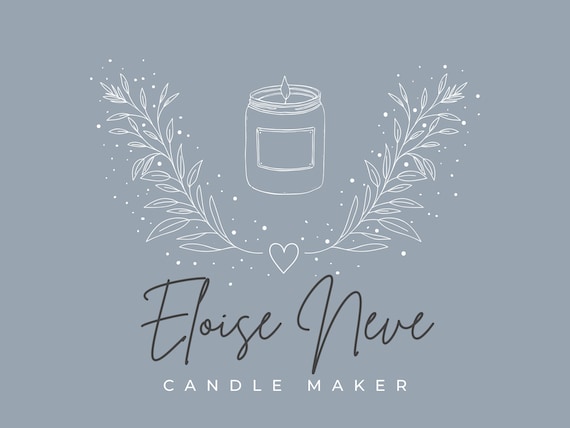The image is a detailed advertisement for Eloise Neve, a candlemaker. Set against a blue-gray background, the center of the image features a meticulously drawn jar candle with a lit wick. The candle's label is blank, emphasizing the focus on the candle's shape and form. Surrounding the candle is a heart at the center, from which sprigs with leaves delicately extend sideways, adorned with tiny white polka dots that scatter elegantly throughout the design. Below the candle, the name "Eloise Neve" is inscribed in elegant cursive, underscored by the word "CANDLEMAKER" in bold, all-caps print. The minimalist yet detailed white outlines give the ad a simple, effective, and artistic appeal.